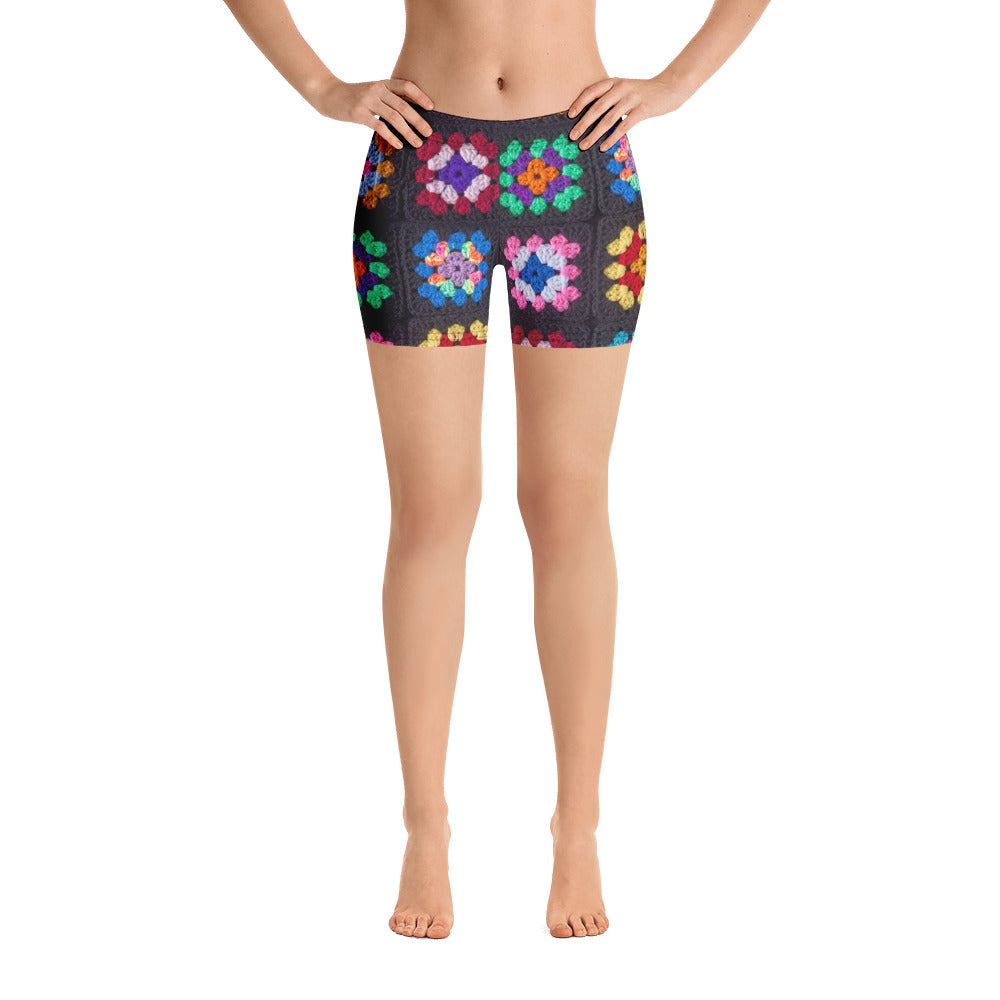This image is a color photograph featuring the lower half of a Caucasian woman, estimated to be around 20 to 25 years old, modeling a pair of tight-fitting, multicolored shorts. The photo is cropped just above her navel, displaying her bare midriff and forearms, with her hands resting on her hips. The woman's legs are bare, and she is standing on her tiptoes on a white background. The shorts, reminiscent of a homemade quilt pattern, feature a vibrant array of colors including green, purple, red, white, blue, and pink, with various flower designs enclosed within squares. The intricate pattern appears as a flat print on the black fabric of the shorts, which are well above the knees. The overall aesthetic is akin to a hand-knit design, adding a whimsical touch to the otherwise stark background.